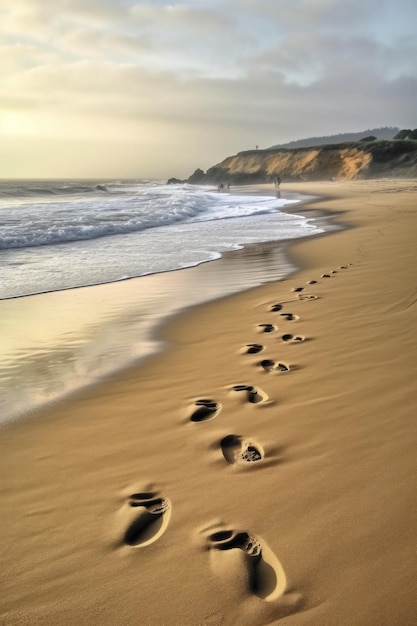In this portrait-oriented image of a serene beach that resembles a painting, the scene showcases a tranquil shoreline with the ocean on the left side transitioning to tan, fine sand on the right. Extending from the bottom center of the image into the distance are clearly visible footprints, though notably, the footsteps appear slightly peculiar, as if two right feet are alternating steps. The footsteps lead towards a distant background where a rocky plateau or small mountain range meets the ocean. 

The beach scene, likely taking place during either sunrise or sunset, is bathed in soft, yellowish light, with the sky displaying a gradient from this warm hue to a darker, cloudier expanse. The ocean waves, capped with white foam, gently lap at the shore. In the far distance, there are faint silhouettes of people walking along the beach, though their details are blurred and indistinct. The backdrop of the mountain range is dotted with sparse vegetation, adding to the natural beauty of the scene.